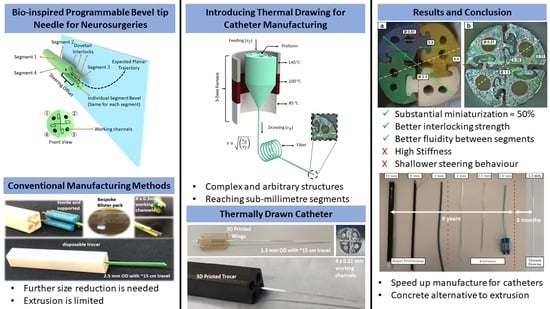The image consists of three detailed instructional panels, each dedicated to explaining different innovations in catheter and needle manufacturing. The left panel features a heading on a blue background, titled "Bio-Inspired Programmable Bevel Tip Needle for Neurosurgeries," and includes a detailed diagram of a green needle with annotations. Below this, there is a section labeled "Conventional Manufacturing Methods" with associated images. The middle panel, also headed on a blue background, introduces "Thermal Drawing for Catheter Manufacturing" with diagrams showing various stages of the process. This section includes images of the equipment used, displaying an aqua-colored plastic funnel with a tube attached. The rightmost panel, titled "Results and Conclusion," showcases various benefits of the newly developed catheters, such as miniaturization, increased interlocking strength, and production efficiency. Collectively, these panels offer a comprehensive look at advanced medical devices designed to improve the effectiveness and speed of neurosurgical procedures.